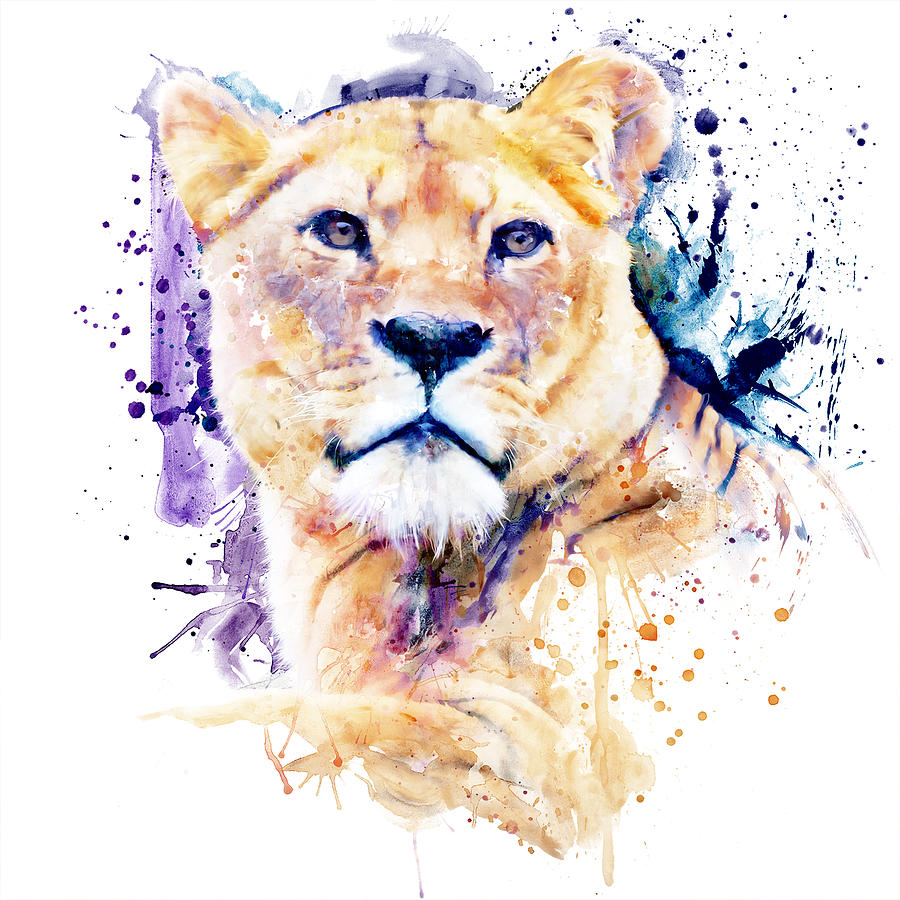This detailed watercolor painting or print features the predominant image of a realistically rendered lion, looking directly forward with a closed mouth. The lion, likely a male due to its prominent mane, has a full head and a portion of its upper torso visible, showcasing detailing such as dark brown eyes, a dark nose, and white surrounding its mouth. Its fur is golden-brown with hints of striping on the back, and the shadowing beneath the chin is accentuated with red and dark purple tones. The background contrasts with more abstract elements, featuring watercolor splotches and dots in various shades of purple and blue, particularly concentrated on the right side of the image. These splashes of color add a dynamic quality, transitioning the piece from a realistic foreground to a more abstract, colorful background. The overall palette predominantly includes purples, dark purples, blues, and the natural golden hues of the lion itself.